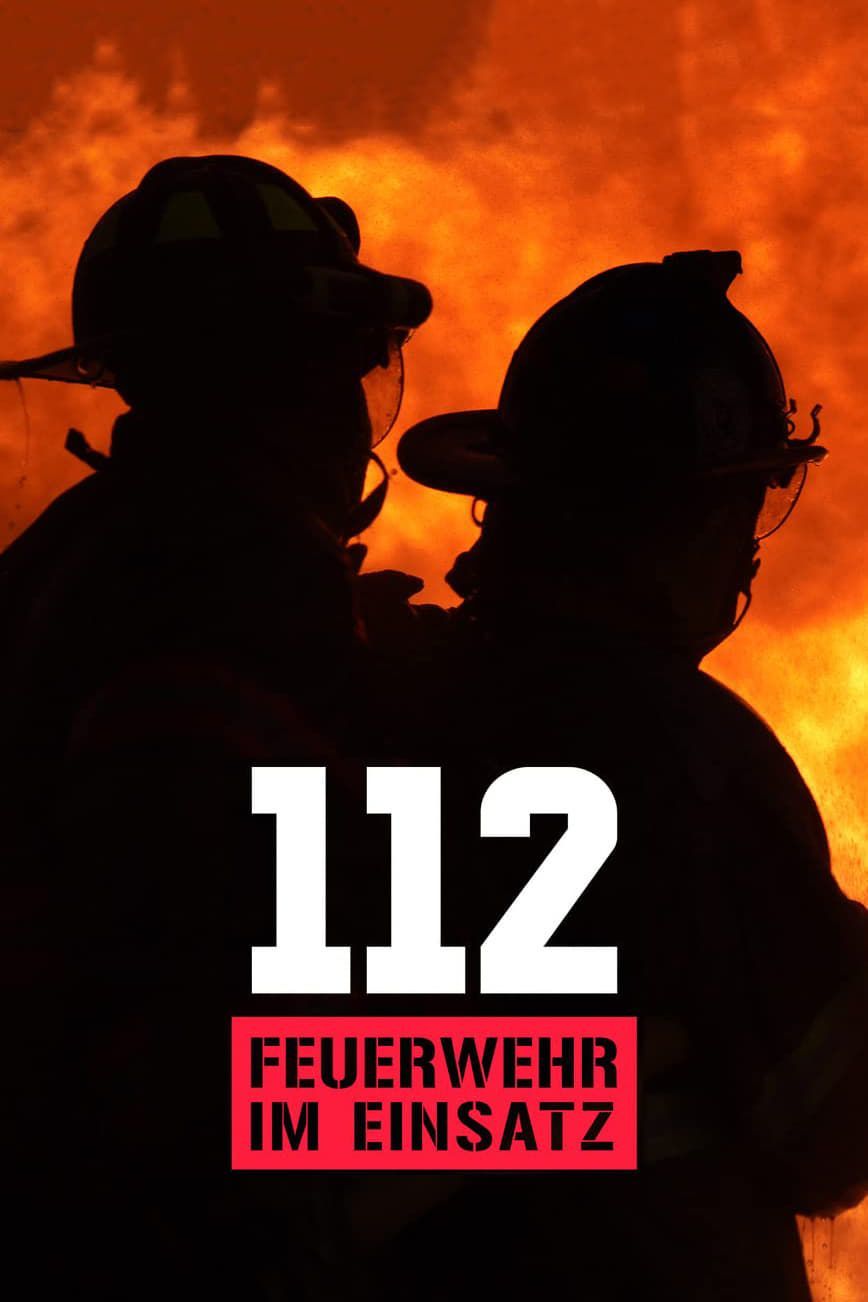This image is a poster featuring two silhouetted figures wearing firefighter gear, prominently positioned against a fiery background of red, orange, and yellow flames. The central part of the poster displays the number "112" in bold white font. Below that, in a red rectangle with black lettering, are the words "FEUERWEHR IM EINSATZ." The contrast between the dark silhouettes and the vibrant flames highlights the intensity and urgency associated with the firefighters depicted. The figures, adorned with helmets, dominate the image, emphasizing their pivotal role in the scene.